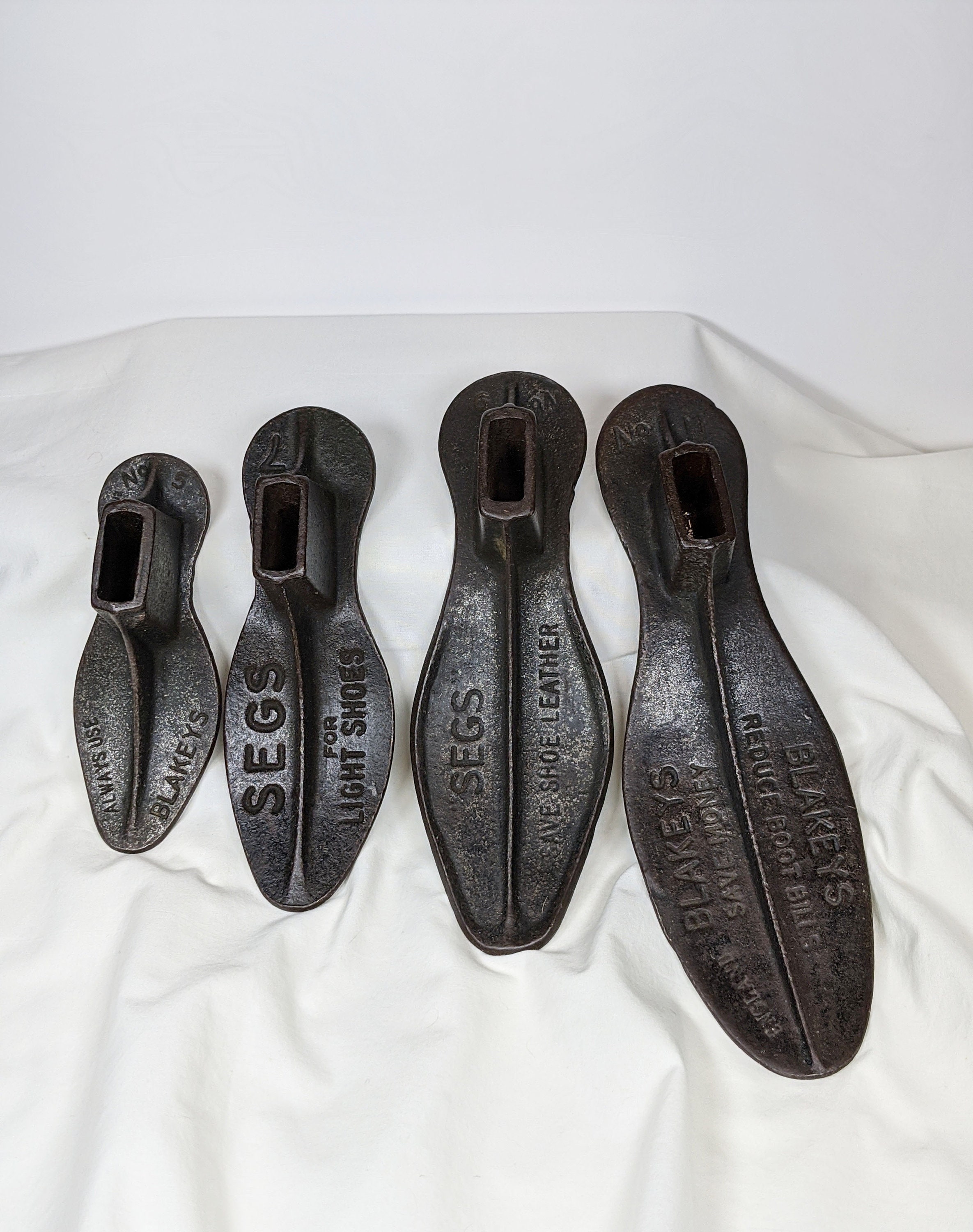This close-up photograph features four cast iron shoe molds displayed on a white sheet with a gray background. The molds are arranged from left to right, smallest to largest, and are designed to either shape shoes or maintain their form. Each mold has a flat base with a taller section at the heel, and they are equipped with slots where bars could be inserted for pressing into leather. The smallest mold is labeled "Always use Blakeys" and is marked with the number five. The second mold, marked with the number seven, reads "Segs for light shoes." The third mold states "Segs save shoe leather," and the largest mold is inscribed with "Blakeys save money, Blakeys reduce boot bills." While the exact numbers on the heel are not entirely legible, these detailed inscriptions suggest these metal objects were crucial tools for a shoemaker.